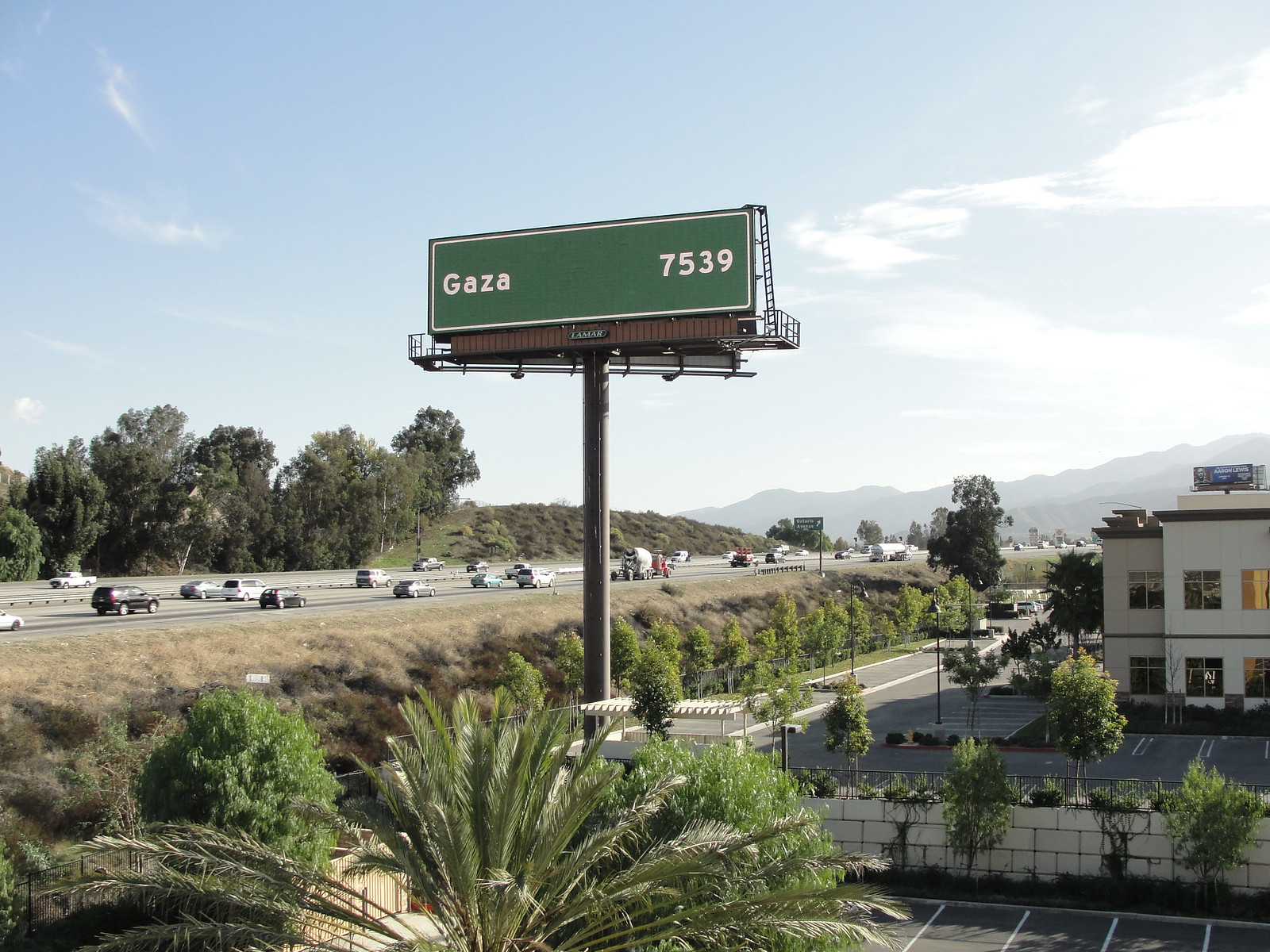This image is likely taken in Israel or the Middle East, as indicated by the "Gaza 7539" sign. The scene features a busy highway populated with multiple cars. In the background, the landscape is dotted with rounded, tall, bush-like trees and grassy, hilly areas. Further down the road, additional signage can be seen, and beyond that, there are mountain-like formations in the distance. In the foreground, before the Gaza sign and away from the highway, tropical plants with a palm tree-like appearance but more bush-like in structure are visible. Across from this scene, there are a couple of buildings which might be either apartment complexes or office buildings, surrounded by a parking lot with a fenced-in area.